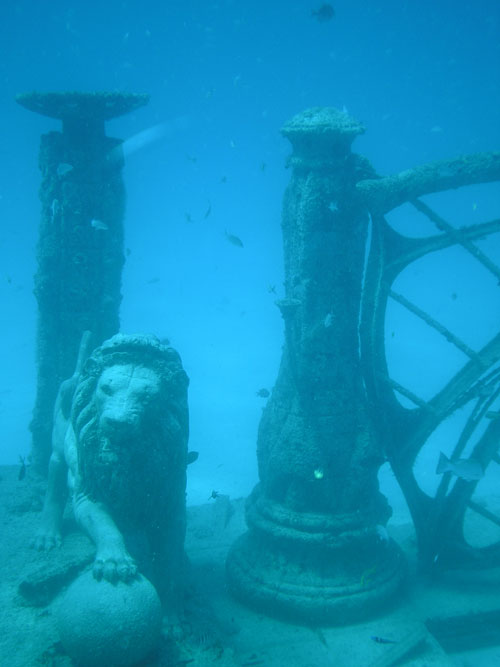The photograph, likely captured using a submersible or through an aquarium glass, displays a mesmerizing underwater scene, predominantly in shades of blue which vary from light to darker hues. At the bottom left corner, a male lion sculpture, carved from stone and appearing weathered from prolonged submersion, confidently holds a round sphere under its left paw. Flanking this majestic figure are two intricately detailed pillars, possibly remnants of an ancient shipwreck or submerged ruins, adding to the historical aura. Small fish swim effortlessly through the scene, emphasizing its aquatic nature and hinting at the passage of time. The light filters gently from the left, illuminating the eerie yet beautiful underwater landscape, giving the entire composition an ethereal quality.